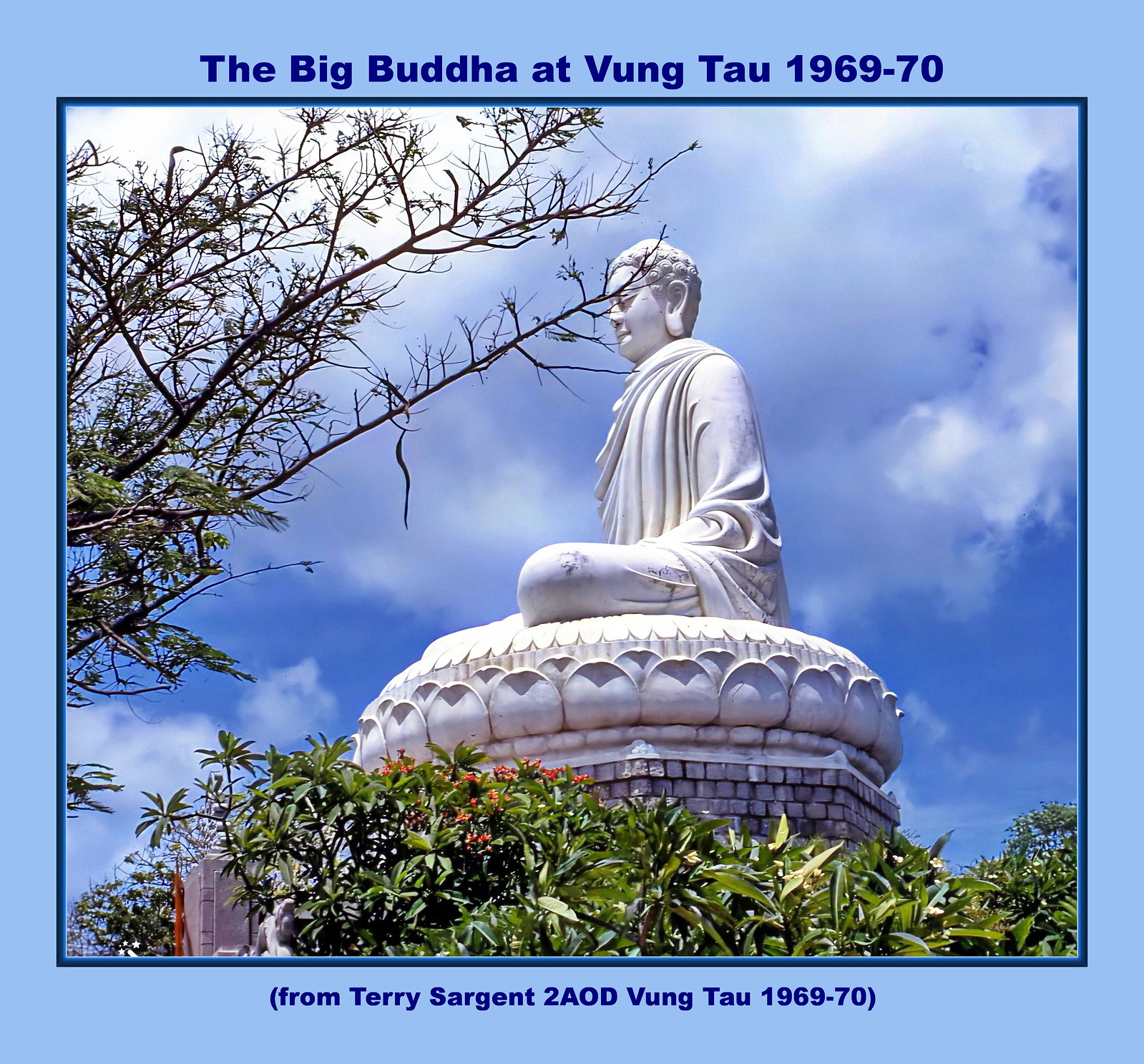The image features a very large, ornate, white statue of a Buddha in a cross-legged or kneeling posture on a cylindrical base composed of gray bricks. The statue, possibly weathered and displaying fine cracks, has a serene expression with closed eyes, suggesting deep contemplation. It wears robes and a head covering. The scene is set against a blue sky with scattered clouds, partially obscured by greenery and tree branches creeping into the frame. The photograph, seemingly taken during daylight hours in a jungle setting with visible trees and shrubs, has a blue border and dark blue text. At the top, bold letters read "The Big Buddha at Vung Tau, 1969 to 1970," and at the bottom, it credits "from Terry Sargent to AOD Vung Tau, 1969 to 1970," indicating it's an older image captured in Vietnam during the late 1960s or early 1970s.